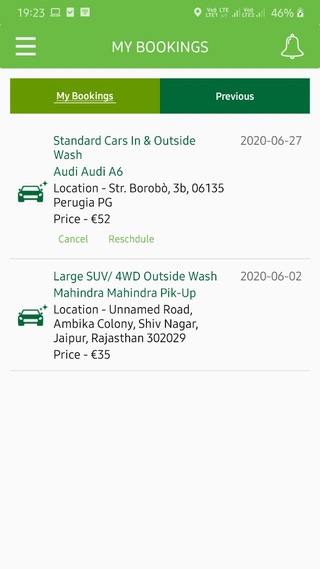### Descriptive Caption 

The image is a screenshot taken from a phone's display, showcasing a travel booking application interface. The layout is as follows:

#### Top Section:
- **Top Bar**: An Apple green bar approximately two inches thick runs horizontally across the top of the screen.
  - On the upper left corner, in white text, it reads "19, 2 3".
  - Next to it, there is a small white icon of a computer, followed by a white box with a green check mark.
  - Further along the top bar, there is another white box displaying the Wi-Fi strength symbol.
  - In the center of the bar, there is a blank space.
  - On the right-hand side of the bar:
    - A white map icon.
    - The text "LTE" in white appears thrice, with the first instance followed by two arrows underneath.
    - The phone signal strength icon shows three out of four bars lit.
    - The battery percentage reads "46%".
    - The battery icon with a black lightning bolt in the middle.
    
#### Middle Section:
- **Header Area**:
  - On the left, there are three horizontal white lines stacked on top of each other.
  - Centered text in white reads "My Bookings".
  - Right of that, an outline of a white bell icon.

- **Tab Section**:
  - The active tab is highlighted in a forest green strip with "My Bookings" in white underlined text.
  - To the right, a darker forest green tab reads "Previous" in white.

#### Booking Details Section:
1. **First Booking**:
   - Green car icon on the left.
   - Text reads:
     - "Standard Cars &" (ampersand symbol)  
     - Underneath, "Wash"  
     - "Audi A6" in green.
   - Location information in black:
     - "Location: Str. BOROBO, 3B, 06135 Perugia PG"
   - Price: "52" preceded by a special currency symbol with two horizontal lines.
   - Action buttons:
     - In green: "Cancel" (left).
     - In white: "Reschedule".
   - Top right of the box: Date "2020-06-27".

   - A thin gray line separates this booking from the next.

2. **Second Booking**:
   - Green car icon on the left.
   - Text reads:
     - "Large SUV - 4WD & Wash" in green.
     - "Mahindra Mahindra PIK-UP" underneath.
   - Location information in black:
     - "Location: Unnamed Road, Ambika Colony, Shiv Nagar, Uttar, Rajasthan, 302029".
   - Price: "35" preceded by the same special currency symbol.
   - Top right of the box: Date "2020-06-02".

Each element and color scheme is designed for ease of navigation and quick information retrieval about the user’s vehicle bookings.